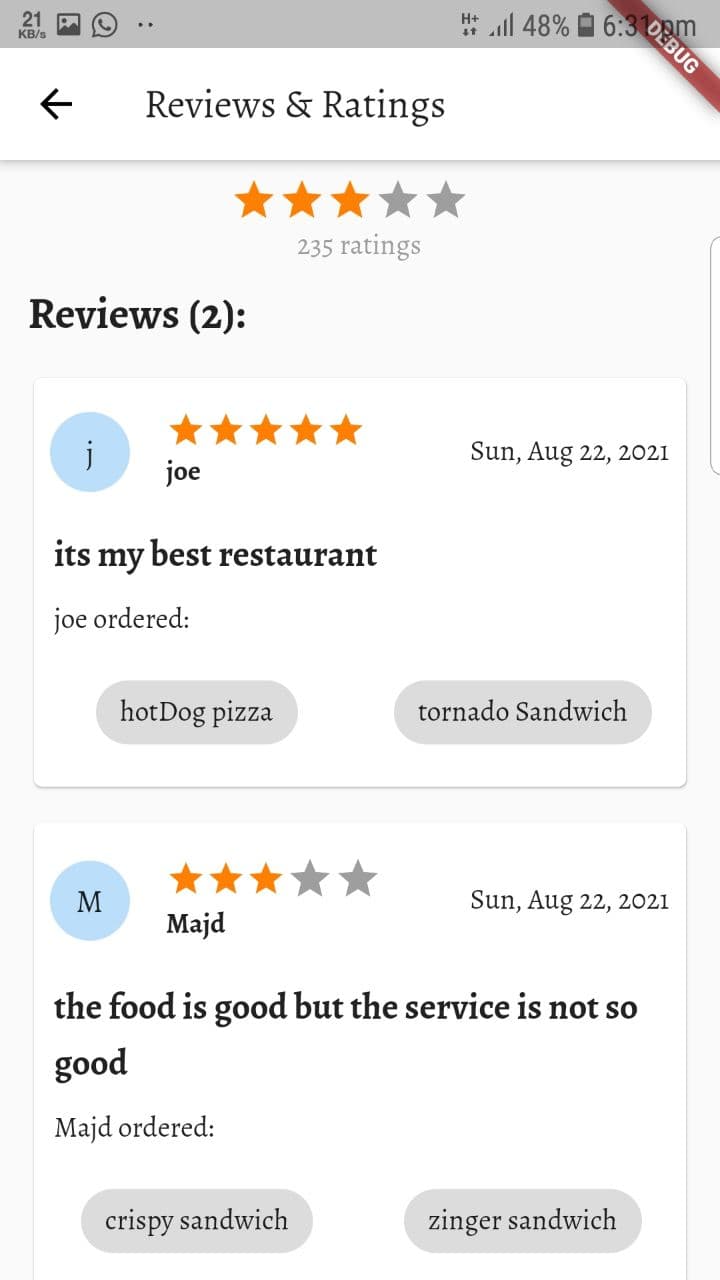**Detailed Caption:**

The image is a vertically oriented rectangle, likely a snapshot taken from a cell phone screen. At the very top, there is a gray banner featuring multiple icons and text in black. On the far left, it displays "21KB/S" followed by a landscape icon, a caption icon with a phone inside, and then two horizontal dots. Towards the right of the banner, starting closer to the center, it shows an "H+" symbol, a four-bar cell phone signal indicator, and a battery life percentage of "48%" accompanied by a battery icon. The time "6:31 PM" is also displayed, with a diagonal red stripe running through it, marked with the word "DEBUG" in white text.

Below the gray banner, on the left side of the screen, there is a left-pointing arrow next to the text "Reviews and Ratings" centered in the middle. Continuing down, a grayish border or line spans the width of the image. Underneath this line, a rating of "3 out of 5 stars" is noted, based on "235 ratings" with the label "Reviews."

Further down, a review by a user named Joe is highlighted. Joe rated the service "5 stars" on August 22, 2021, and commented, "It's my best restaurant." Joe mentioned that he ordered a hot dog pizza and a tornado sandwich.